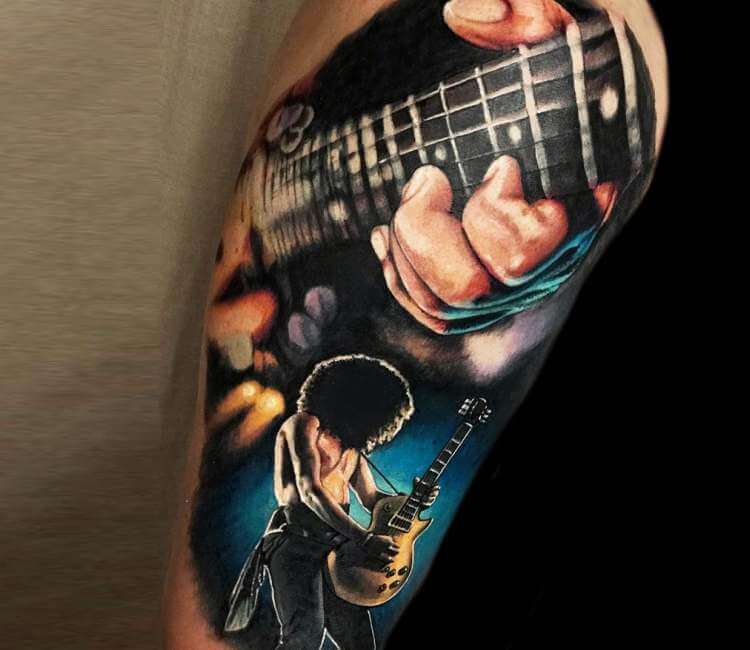This image appears to be a close-up tattoo, most likely located on someone's upper arm or shoulder. The tattoo art vividly portrays a shirtless man with an afro hairstyle, playing a yellow and black electric guitar. The top of the tattoo focuses on a close-up of the fingers making chords on the guitar. The figure's face is obscured, showcasing only the outline of his prominent hair and body. He is depicted wearing black or gray jeans, with a hanky visible in the back pocket. The color palette of the tattoo features deep blues, blacks, yellows, and golds, with the right side of the tattoo showcasing a black background, while the left side displays a beige or tan pattern. The intricate details and use of color bring the image to life, creating a striking piece of body art.